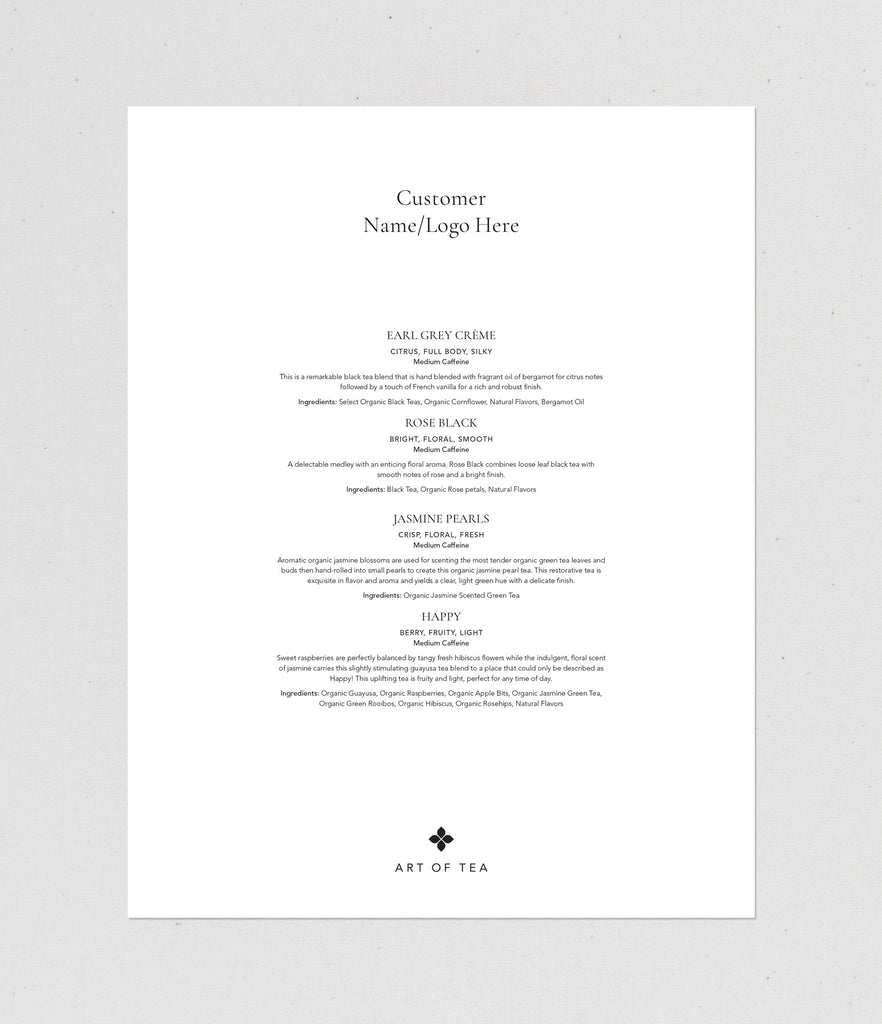In the image, a white piece of paper resembling a menu is set against a blue background. At the top, it prominently features the text "Customer Name/Logo Here" in centered blue letters. Below this header, the menu is divided into four sections, each with detailed descriptions. The first section is "Earl Grey Cream" described as citrus, full-bodied, and silky with medium caffeine, containing select organic black teas, organic cornflower, natural flavors, and bergamot oil. The second section, "Rose Black," is characterized as bright, floral, and smooth with medium caffeine, featuring black tea, organic rose petals, and natural flavors. The third section, "Jasmine Pearls," noted as crisp, floral, and fresh with medium caffeine, consists of organic jasmine-scented green tea. The final section, "Happy," described as fruity and light with medium caffeine, includes organic raspberry, organic apple bits, organic jasmine green tea, organic green rooibos, organic hibiscus, organic rose hips, and natural flavors. At the bottom, a black four-petal flower logo accompanies the text "Art of Tea." The entire menu text is centered, consistent, and the finer details are dense and closely spaced.